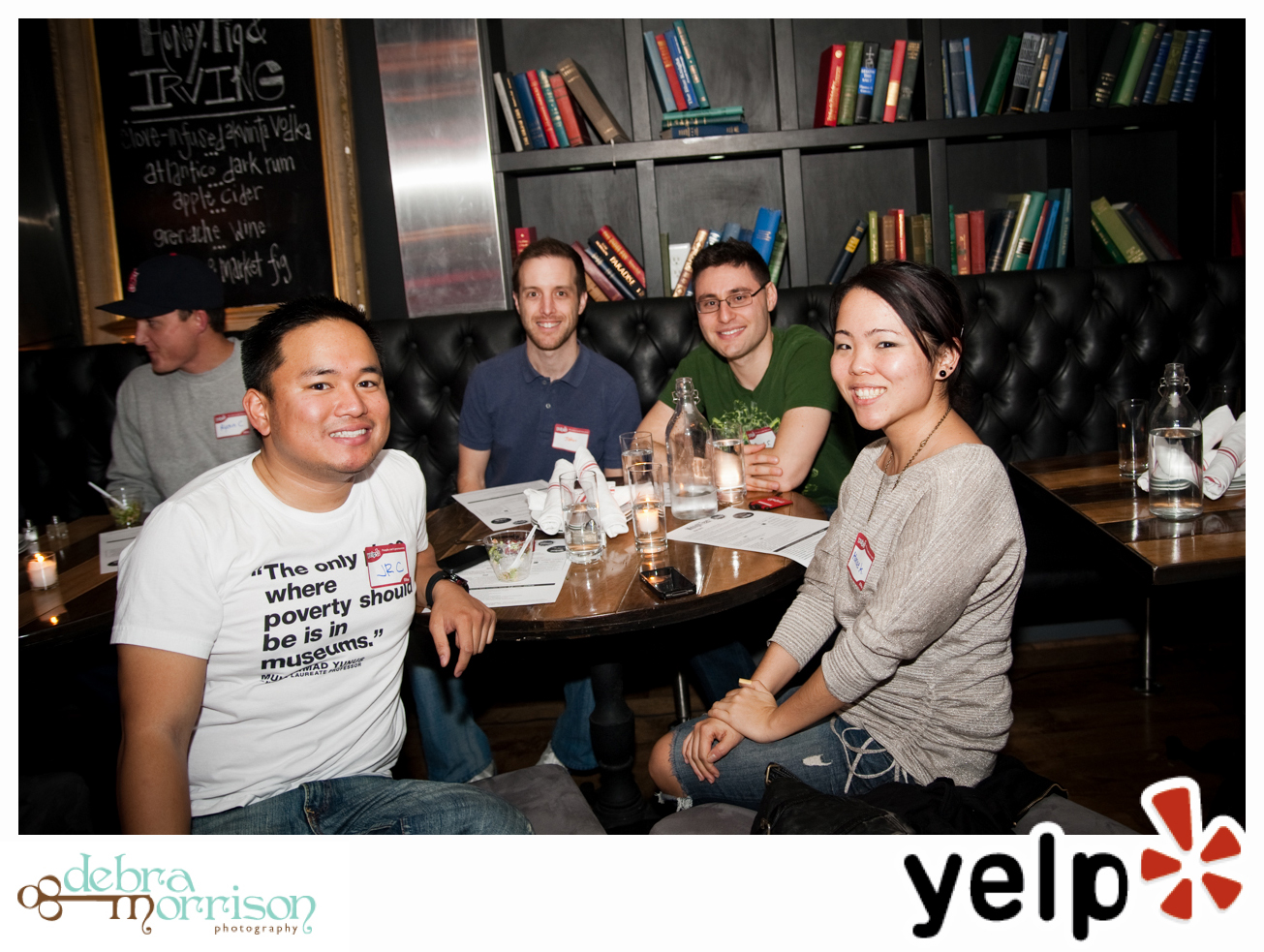In this detailed photograph, a lively scene unfolds in a cozy café or restaurant, featuring a round table with four people engaging warmly. At the round table, starting from the right, is a cheerful young woman with long dark hair, wearing a long-sleeved shirt and jeans with a noticeable hole. She is smiling broadly. Next to her, on the left, is a man dressed in a white t-shirt emblazoned with the slogan, "The only place where poverty should be is in museums," partially obscured by a white name tag on his left side. He has short black hair and is also smiling. Two other individuals at the same table, both with dark hair, are facing the camera; one wears a blue shirt and is positioned on the left, while the other, in a green t-shirt, sits on the right.

To the left of this group, another person is partially in view, sitting on a black bench with a black backrest. This individual sports a dark hat and a gray shirt, also with a name tag on the left side of their chest. This person appears to be looking slightly away from the camera.

The backdrop of this image is filled with character: a black bookshelf with small cubbyholes stuffed with books of various colors—including yellow, red, and multicolored volumes—adds to the ambiance. On the far left, a black board with white letters is faintly visible, and a chalkboard with unreadable writing adds a rustic touch to the setting.Overall, all five people in the photo are wearing name tags, highlighting a social or communal gathering in a comfortable and welcoming indoor environment.